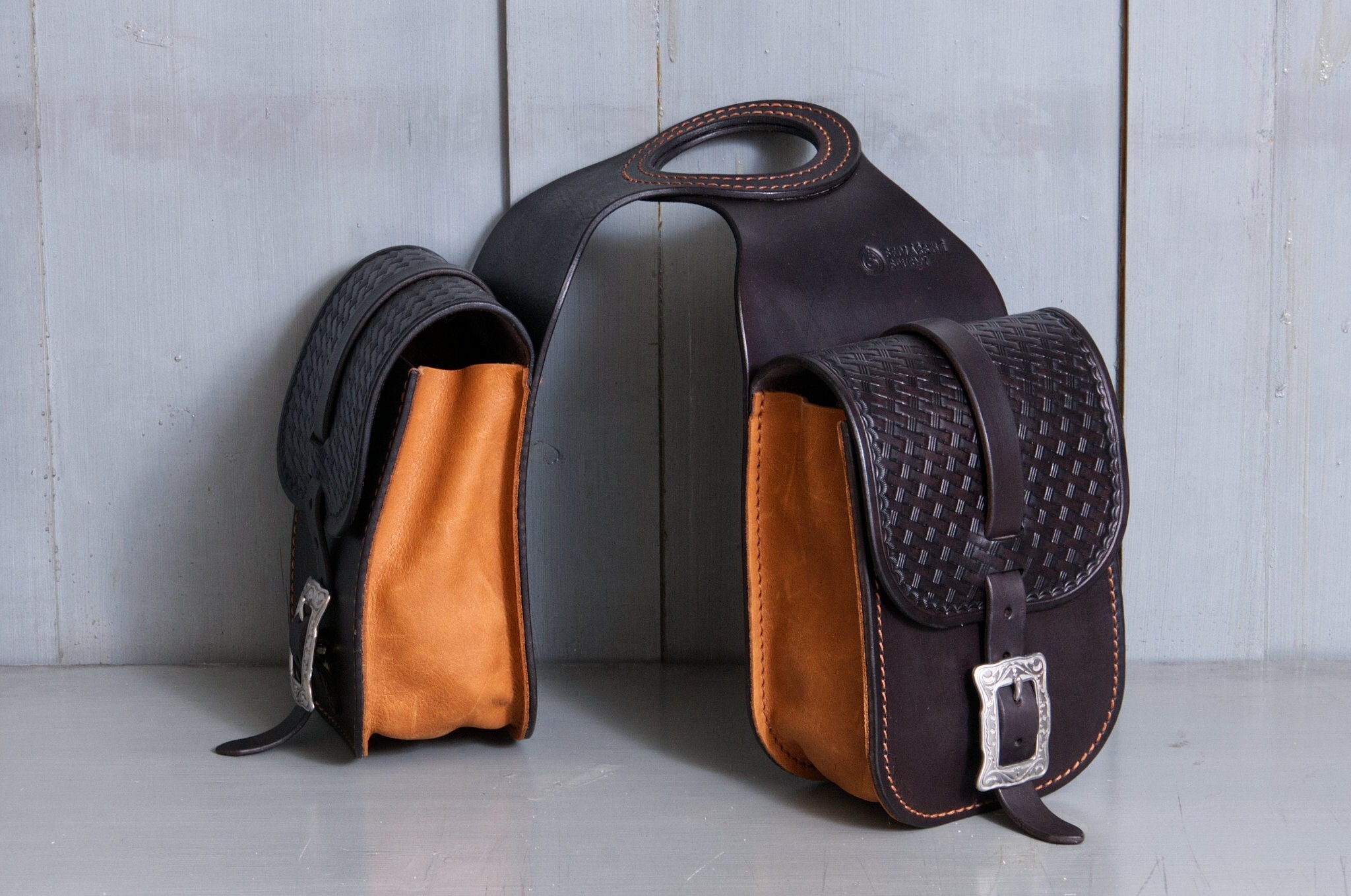This image depicts a set of leather saddlebags designed for use on a horse. The saddlebags, crafted from high-quality leather, feature a combination of dark brown and orangish-brown hues. Each side of the saddlebags has a darker woven flap, secured with a silver buckle and attached by a strap that forms a cohesive design with the rest of the bag. The main body of the saddlebags is secured to a saddle horn via a large hole at the top. Intricate orangish-brown stitching runs along the edges, adding a touch of contrast and detail. The saddlebags are displayed against a grayish-white, smoothly polished surface with a matching white and gray wall in the background. This highlights the craftsmanship and functional design of the saddlebags.